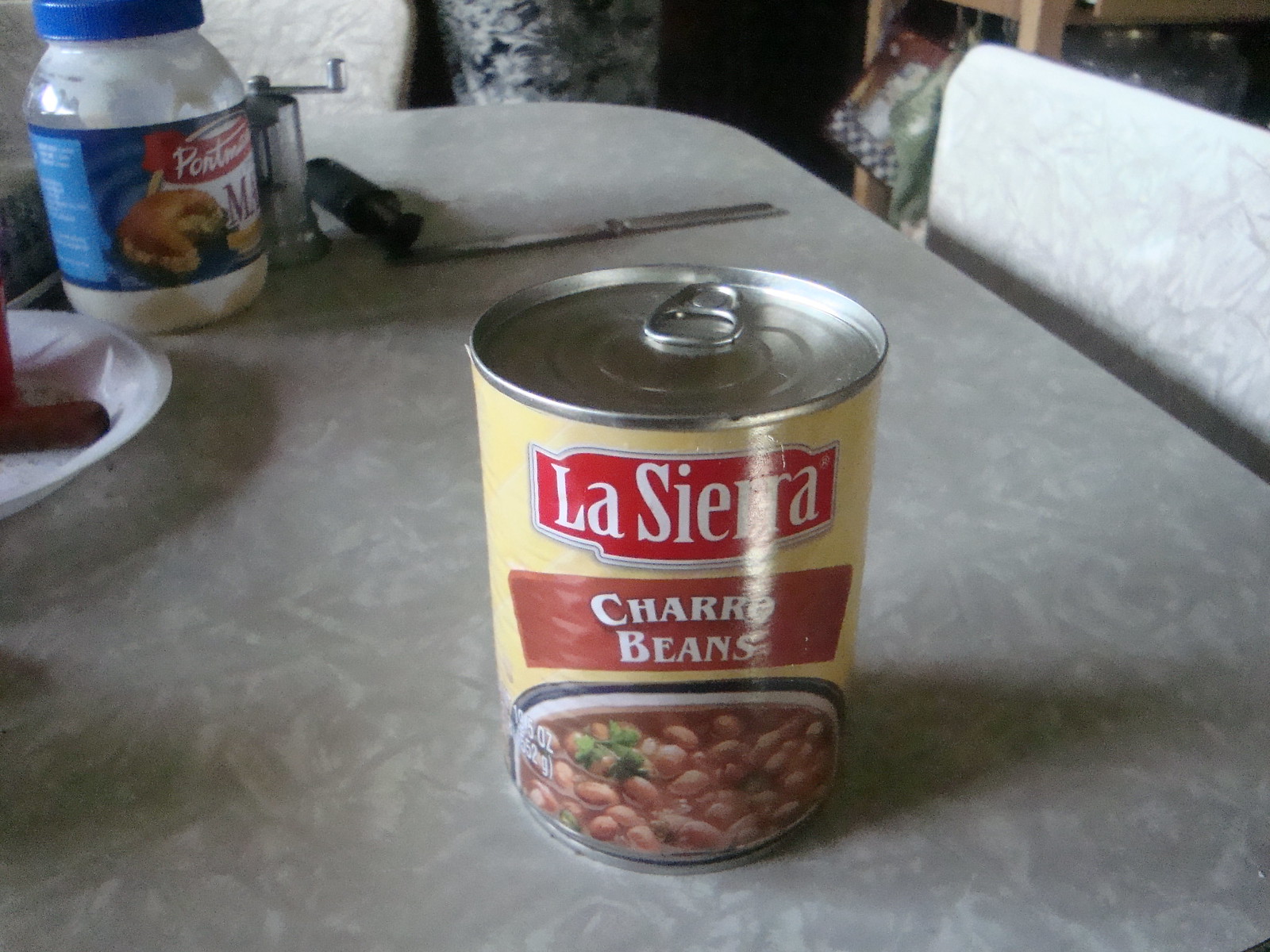The image is a detailed snapshot of a kitchen table scene. Dominating the foreground is a can of La Sierra Charro Beans, featuring a distinctive label with white text on a red, squared-and-rounded logo. The rest of the label transitions to a beige color, and prominently displays a picture of beans in a white pot with a black rim. Surrounding the can on the gray table are various everyday items, including a jar of mayonnaise with its label turned away, a butter knife, and a plastic or styrofoam plate. Positioned behind the can, there appears to be a hot dog poking out of the plate. A chair matching the table's color is partially visible to the right, suggesting a casual dining setup within a kitchen setting.